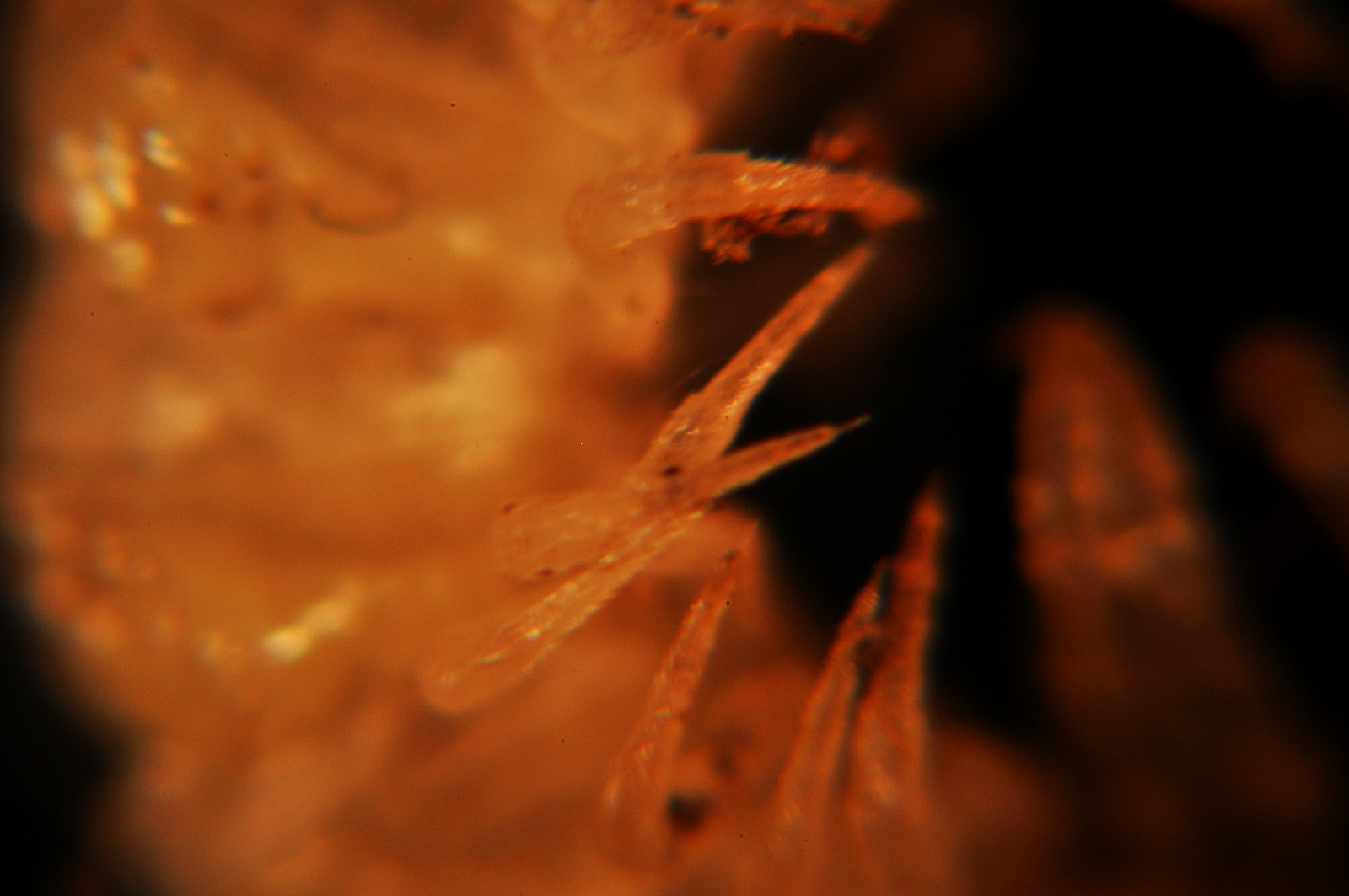This image depicts a highly magnified close-up photograph of the underside of an insect, possibly a caterpillar. The insect's body is colored in shades of reddish orange to yellowish orange, starkly contrasted against a solid black background. The magnification reveals sharp, claw-like legs or hair-like structures emerging from its abdomen, creating a somewhat creepy and eerie visual reminiscent of looking through a microscope at a bacteria or virus. Despite the enhanced detail, the image remains slightly blurry, lending a vague and somewhat unsettling impression of the insect's anatomy. The vivid colors and the positioning of the legs make the creature appear almost as if it were in motion, with a hint of a possible tail visible in the background.